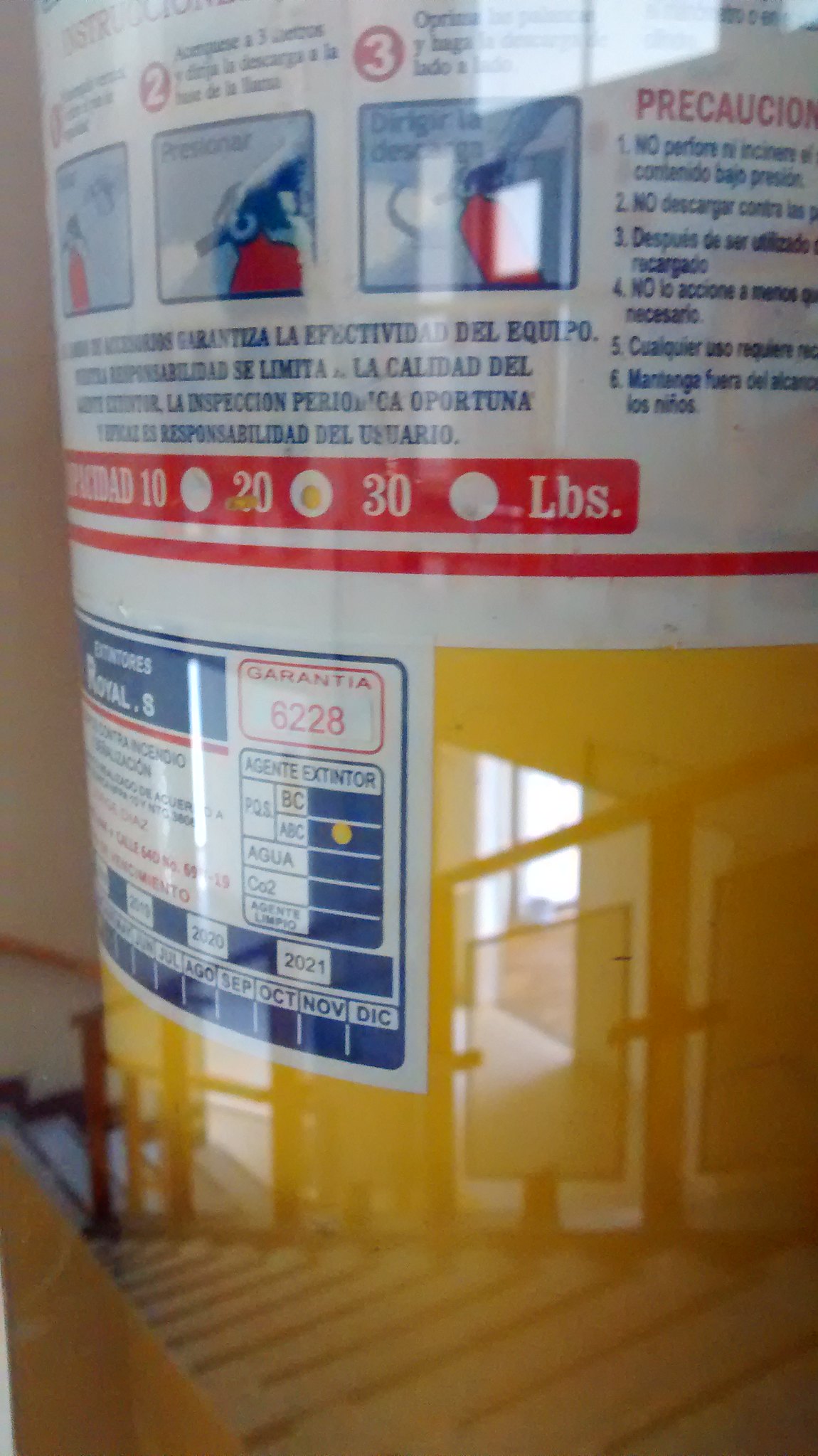The image features a yellow fire extinguisher with detailed labeling. At the top of the extinguisher, there is a three-step instructional guide in red, illustrating how to use the device. The extinguisher itself contrasts with the red infographic by being entirely yellow. Additional text, which appears to be safety and precautionary information, is prominently displayed in Spanish. The overall layout and instructions suggest that the device is indeed a fire extinguisher, despite the initial ambiguity.